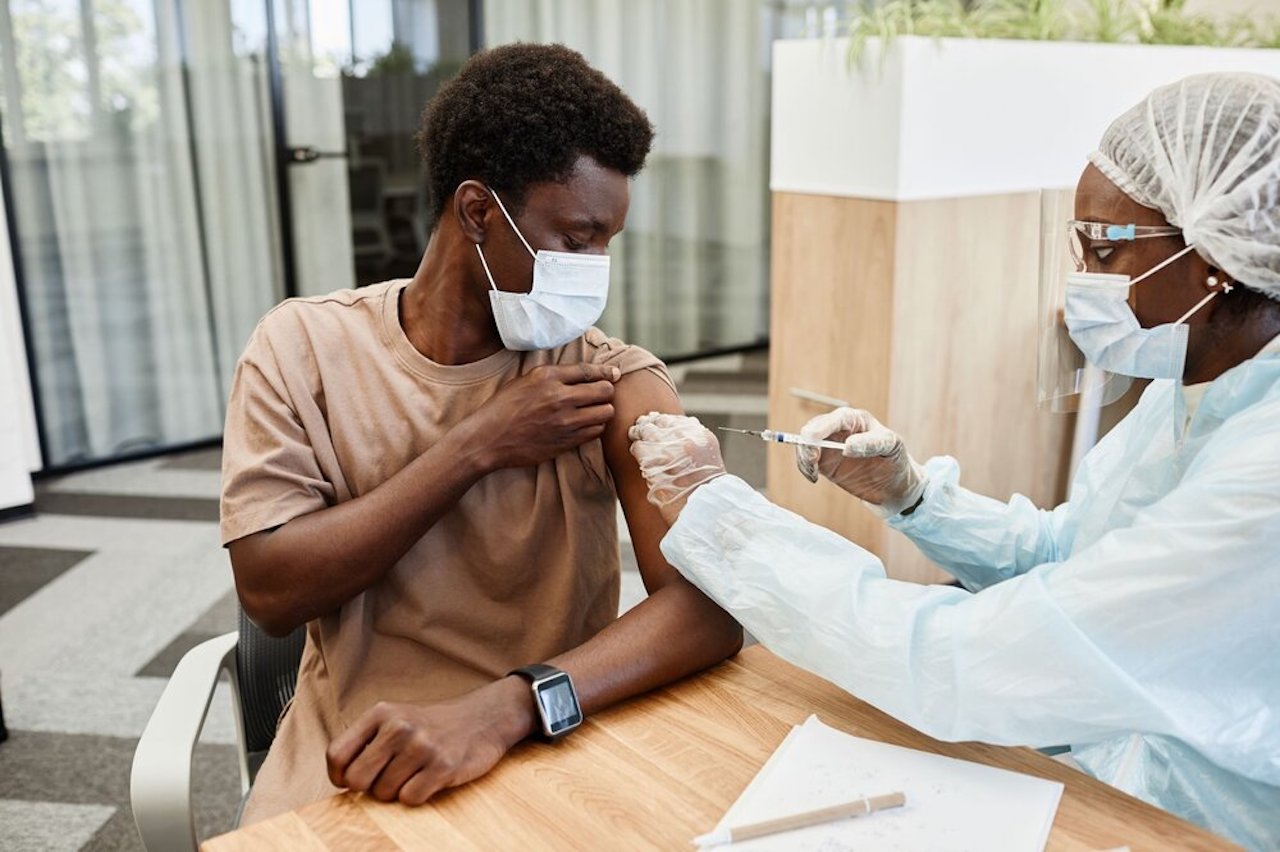This color photograph captures a detailed scene of a young African American man, probably in his twenties, receiving a vaccination shot from an African American woman, likely in her thirties to fifties, in a medical office setting. The man sits on the left, wearing a brown t-shirt with his sleeve rolled up and holding it with one hand, equipped with a wristwatch and a protective face mask. He rests his elbow on a light brown table that has a piece of white paper and a pen on it. The female medical personnel, positioned on the right, is dressed in a protective jacket, face mask, glasses, and a white hair net. She is poised to administer the shot with a syringe. The room is indicative of a clinical environment, complete with walls, curtains, doors, and windows in colors including brown, light blue, beige, gray, and white. The subtle details of the scene add to its authenticity, emphasizing the seriousness and precision involved in the medical procedure.